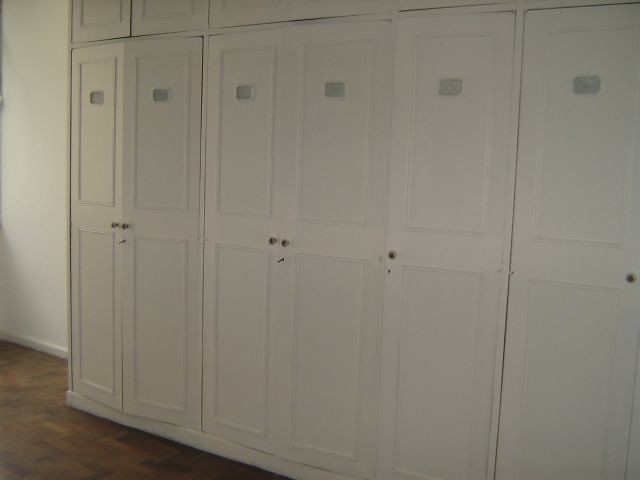The image showcases a large, old-style white wardrobe that occupies the entire right side of the frame. The wardrobe is positioned on a brown hardwood or parquet floor, visible in the bottom left corner of the image, and is set against a white wall, seen in the upper left corner. The wardrobe appears to have two tiers, with the bottom tier comprising at least six tall doors adorned with small circular knobs positioned near their inner edges. These white doors feature small gray rectangles at the top. There are likely more doors extending off the right side of the image. The doors on the left end of the wardrobe are slightly ajar, suggesting a functional, everyday use, possibly to store clothes or other items.